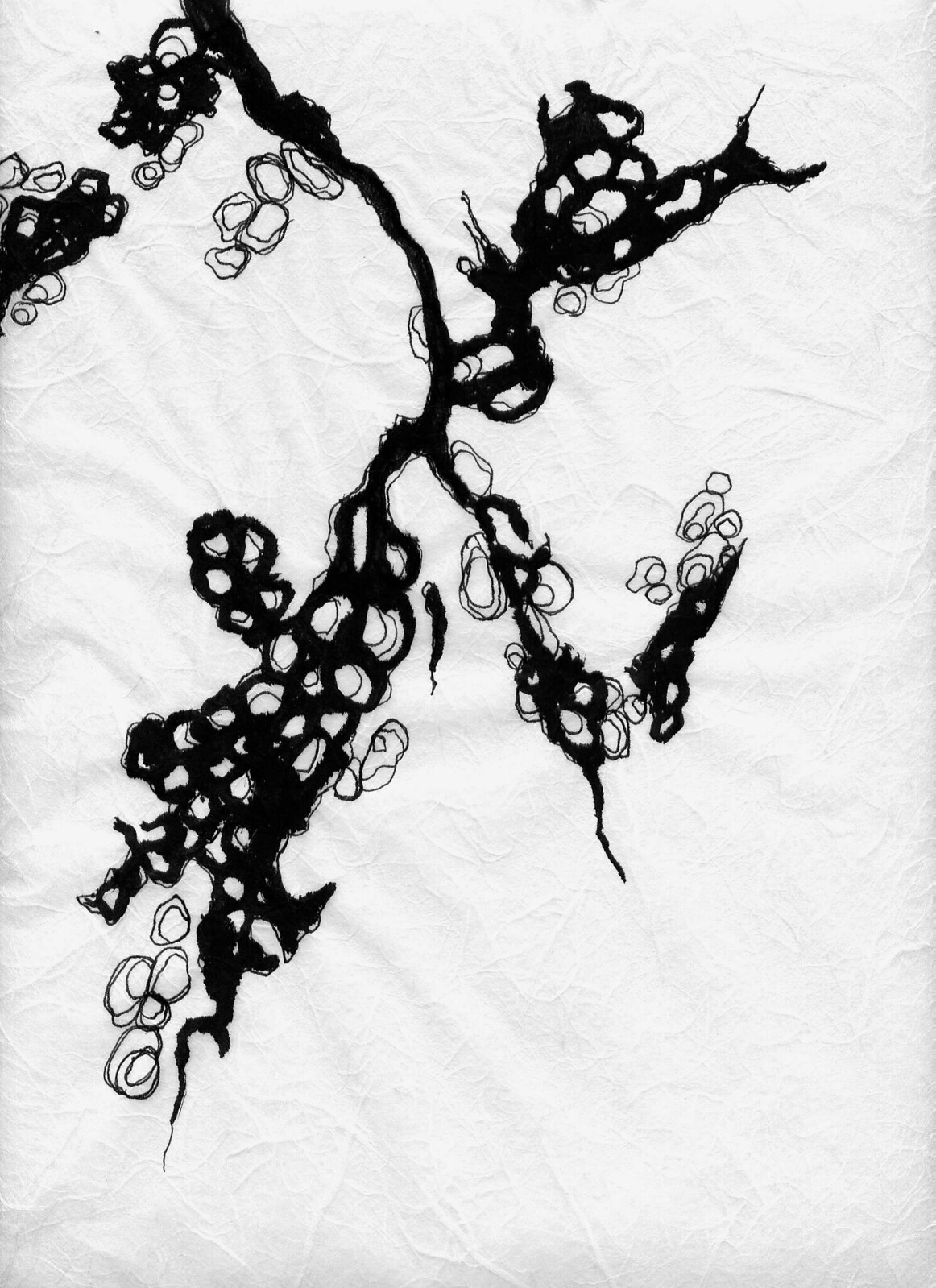This photograph showcases an abstract drawing rendered in black ink or marker on a white cloth or paper. The white surface, which exhibits some wrinkles and creases, acts as a textured backdrop for a complex design that spans from the upper left to the lower left side of the composition. Central to the drawing is a prominent vertical line from which numerous irregular branches radiate, forming various imperfect circles and loops reminiscent of organic growth patterns or plant roots. The black design varies in thickness, with some lines resembling thin threads and others appearing more like thick yarn, creating a dynamic interplay of shapes that evoke different interpretations, including dragon heads and abstract scribbles. The overall effect is a rich and intricate pattern that emphasizes the contrast between the stark black lines and the white, textured background.